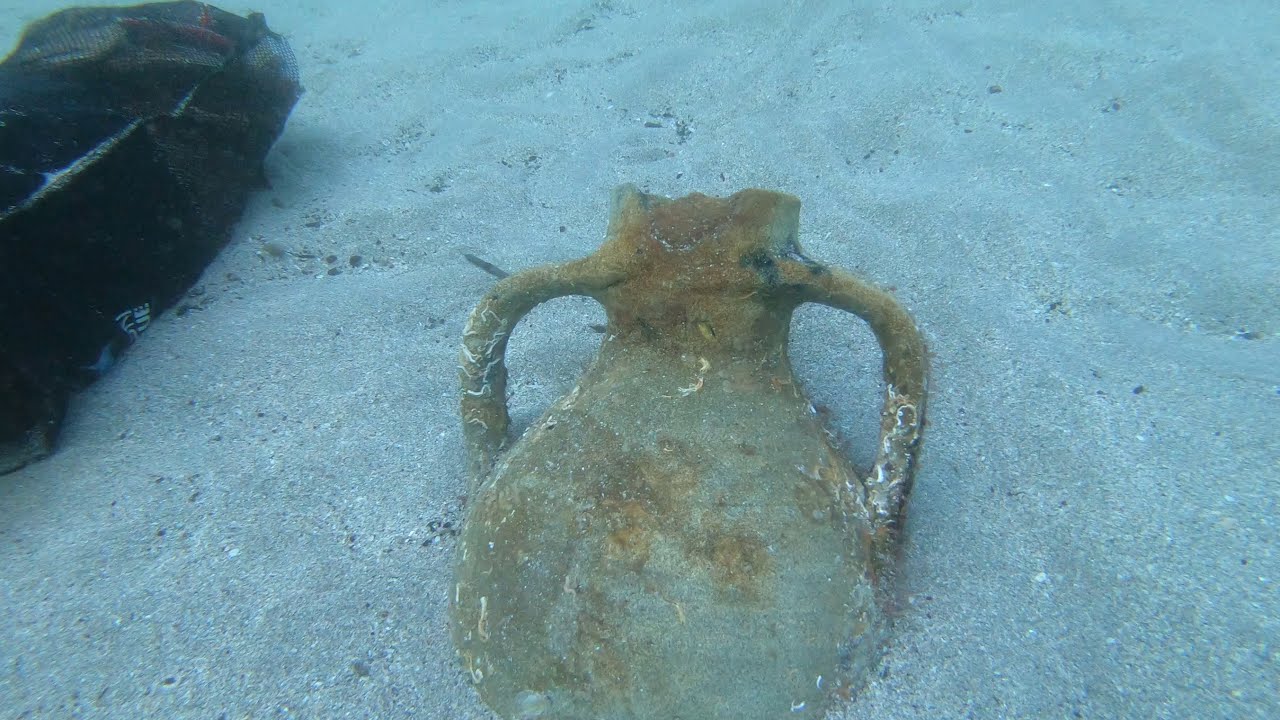The image depicts an ancient, pear-shaped urn that appears to be submerged underwater, enveloped in a bluish tint characteristic of deep-sea scenes. The urn, crafted from either ceramic or stone, features a narrow neck that expands into a wide, bulbous bottom, and is adorned with two handles extending from the neck to the base. Faded and discolored from prolonged exposure, patches of oxidized orange and white coral-like tendrils adorn its surface, giving it a rustic and weathered appearance. The urn is partially buried in what seems to be a fine, bluish-gray sandy seabed mixed with small, crushed shells. In the upper left corner of the image, an old, black fishing net, covered in brown algae, adds to the underwater ambiance, invoking a sense of long-term submersion and forgotten relics at the bottom of the ocean.